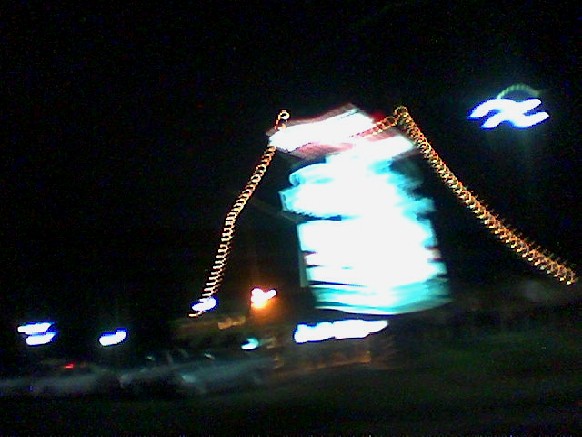A blurred and abstract nighttime photograph appears to have been taken in motion, likely from a moving vehicle, capturing a parking lot scene. The centerpiece of the image is a large, neon sign situated on the middle left, taking up about a third of the photograph. Due to the motion, the sign's bright blue and white lights blur into amorphous halos. Above this large sign, there is a smaller, bright red and white light. Two downward-angled, lighted cables extend from either side of the image. In the top right corner, an 'X' shape encompassed by a green, half circle can be faintly discerned against the dark sky backdrop. The bottom of the image reveals at least four parked vehicles, their colors indeterminate in the dim light. To the right of the main sign, a smaller, illegible sign written in script style can be seen. The bright lights and composition evoke an impression of a bustling location, possibly a shopping complex or hotel, reminiscent of a Las Vegas scene.